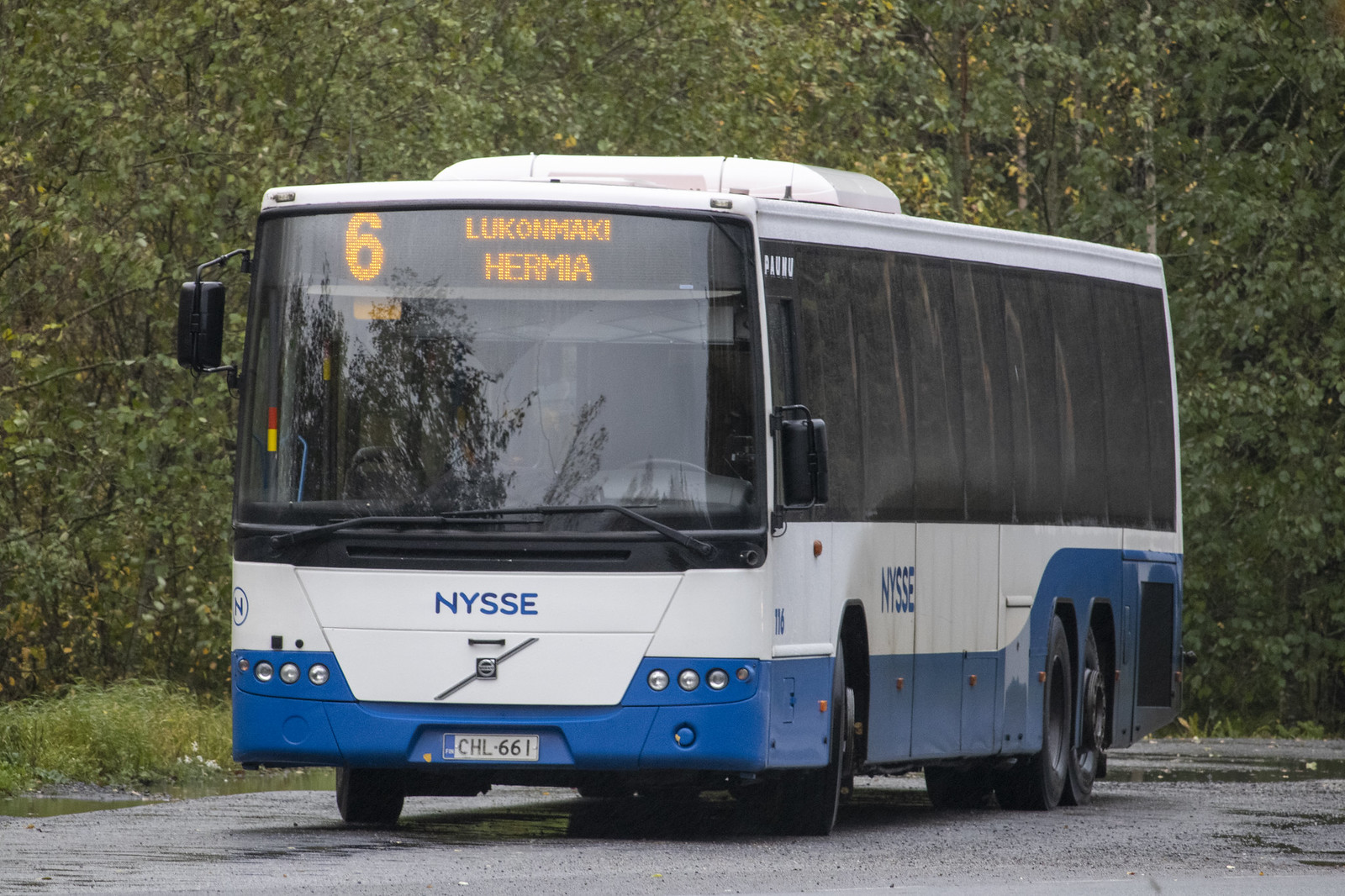The photograph depicts a blue and white city bus, prominently positioned at the center of a gray concrete roadway. The bus displays dark, tinted windows, with its left-hand side showing three visible wheels. Distinctive blue trim accentuates the primarily white exterior, running along the bottom side panels and around the headlights.

Marked on the front of the bus, beneath the driver’s window, is the name "NYSSE" in blue lettering, accompanied by the license plate "CHL-661." An electric billboard at the top front of the bus displays a large number "6" in yellow, followed by “LUKONMAKI” and “HERMIA,” both spelled out in the same yellow font. 

The bus appears to be part of a European public transportation system, inferred from the style of the license plate and the language on the signage. The surrounding environment features densely populated green trees on either side, reinforcing the bus's predominant position in an open, possibly urban or suburban, landscape.